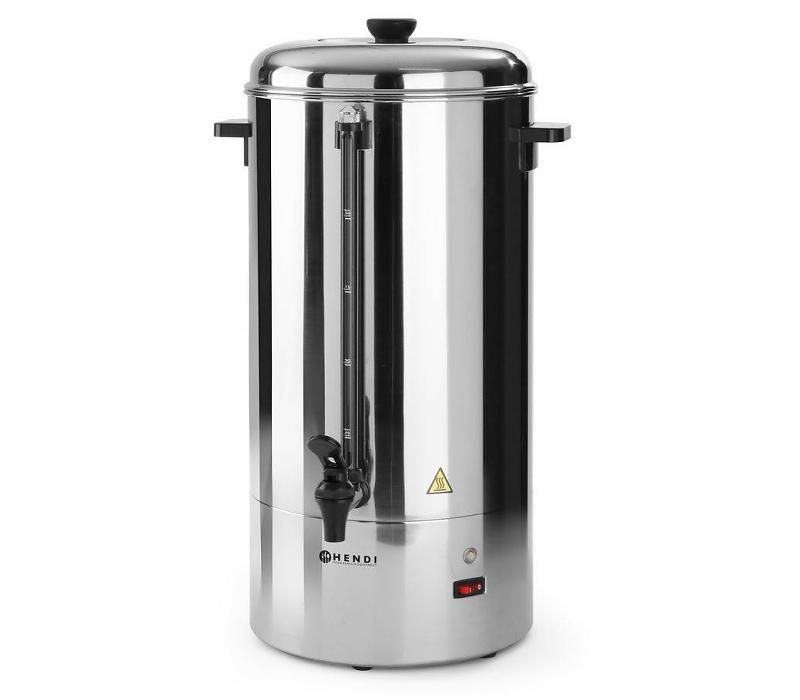This image features a tall, silver coffee carafe or percolator designed for buffet settings or large gatherings. The carafe, photographed against a white background, has a cylindrical shape and is equipped with small black handles on either side for easy portability. The lid features a black knob handle for safe handling. On the front, there is a black dispenser with a window to indicate the liquid level inside. The carafe prominently displays the brand name "HENDI" (H-E-N-D-I) in black text. Above the dispenser, a small yellow triangle with swirly lines symbolizes heat. At the bottom of the carafe, a red rectangular switch is labeled with "off" and "on" for power control. Notably, the carafe is new, with a shiny, polished finish, ideal for serving hot water, coffee, or tea at meetings or events.